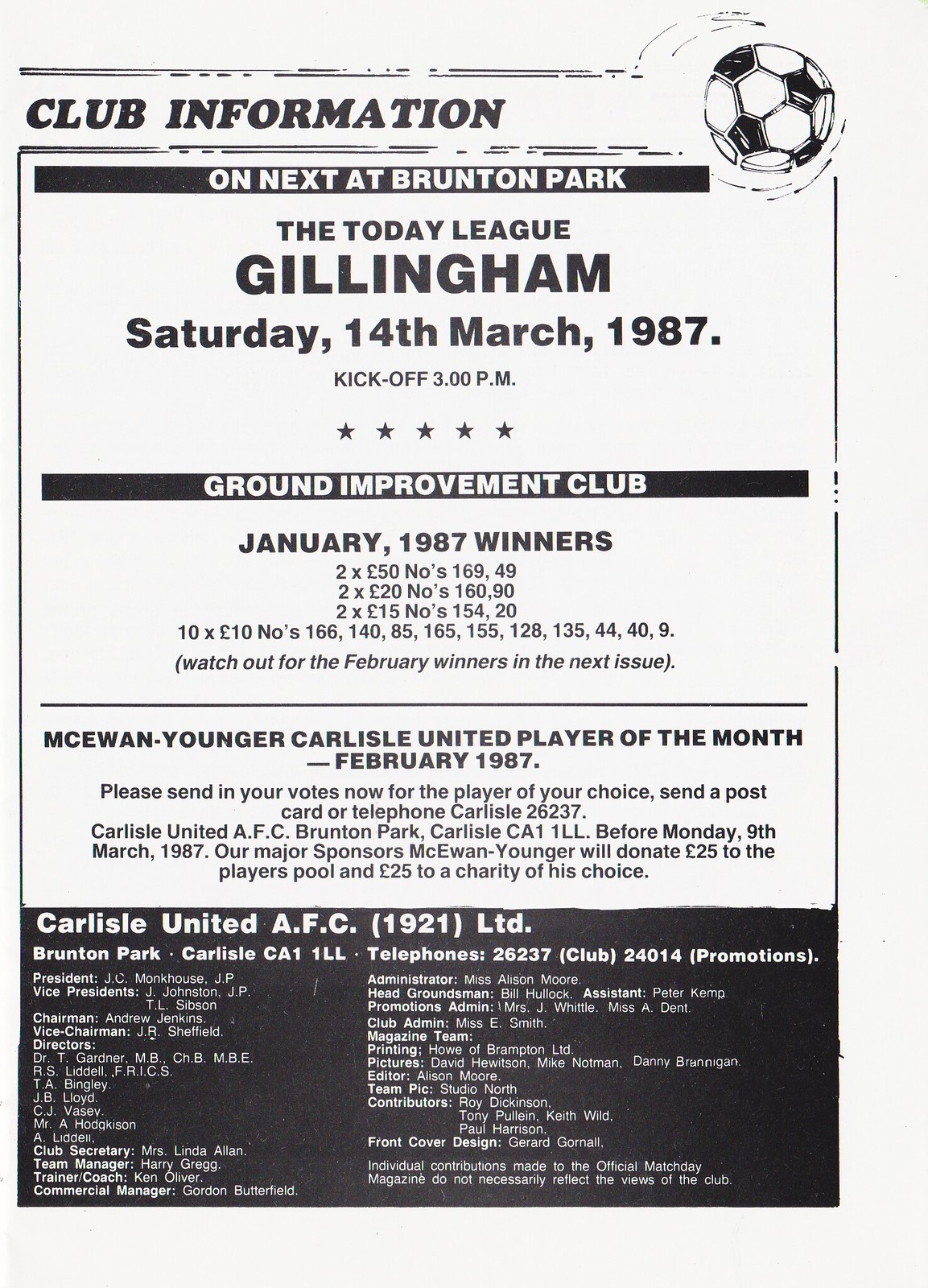The image is a black and white flyer detailing a football event. At the top, it prominently displays "Club Information" in bold black letters. In the upper right corner, there's a graphic of a black and white soccer ball. Below, it announces the "Today League" match between Brunton Park and Gillingham, scheduled for Saturday, 14th March 1987, with kickoff at 3pm. The flyer includes details about a Ground Improvement Club event, mentioning January 1987 winners who received a prize of two $50 Euro notes, indicated by numbers 169 to 49.

In the lower section, it highlights MCE Juan Younger as the Carlisle United Player of the Month for February 1987 and urges fans to send in their votes via postcard or telephone to Carlisle 26237. The bottom part of the flyer contains the club’s full name, "Carlisle United AFC 1921 LTD," along with their address at Brunton Park, Carlisle GA1 1LL. There are also contact numbers and credits for the magazine team, including information on the printing, pictures, editor, and contributors. The entire flyer is designed in black and white, with the black text standing out against a white background, giving it a clean and formal appearance.